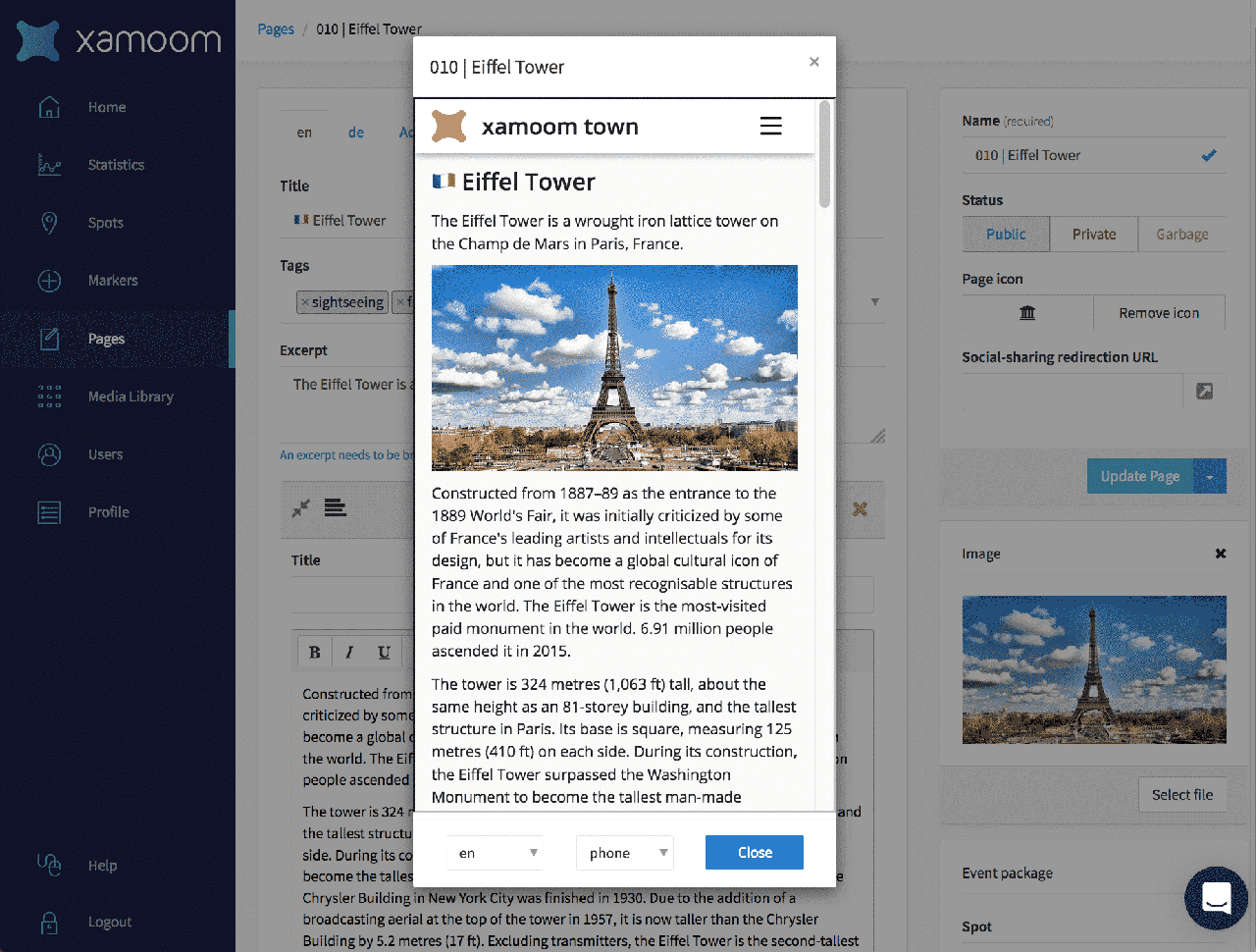This image showcases a pop-up window from the XAMOOM website. In the upper left-hand corner, the title "XAMOOM" is visible, and below it sits a vertical menu. The pop-up window, primarily white in color, contains detailed information about the Eiffel Tower, prominently displayed on the right. The top-left corner of the pop-up window features the identifier "010." Below it, the title "Eiffel Tower" is presented, followed by the subtitle "XAMOOM Town." Further below, the title "Eiffel Tower" is reiterated. A descriptive blurb begins with "The Eiffel Tower is a wrought iron lattice tower on the Champ de Mars in Paris, France." Additionally, the window includes a small photo capturing an aerial perspective of the Eiffel Tower, set against a backdrop of a cloudy sky, displaying the full structure in its entirety.